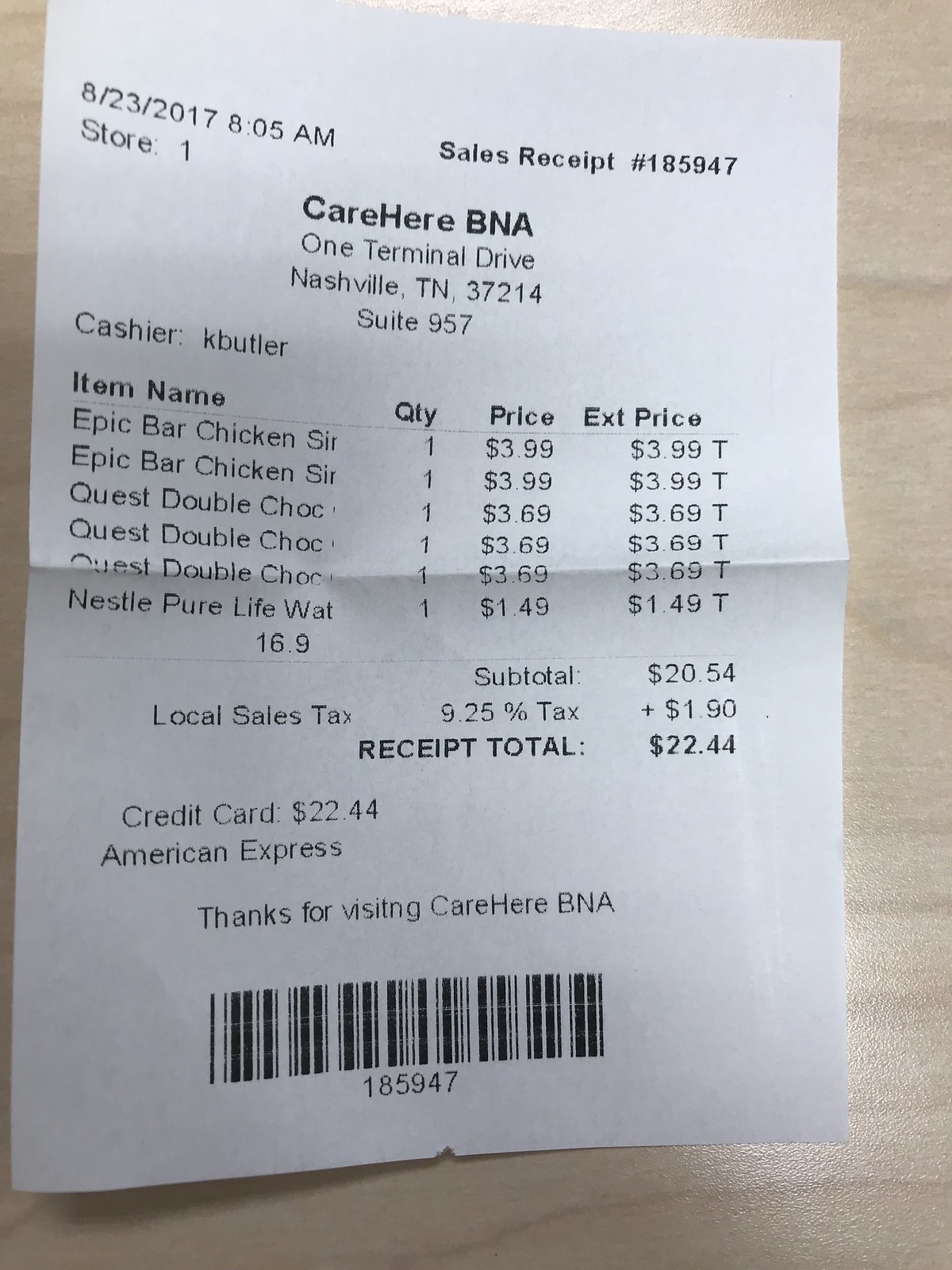The image depicts a detailed takeout receipt, prominently displayed on a light wood surface with visible grains, reminiscent of an ash blonde or light pine finish. The receipt itself is white with black text and occupies the majority of the image. At the top left corner, the date and time are noted: 8-23-2017, 8:05 AM, with the store number listed as 1. To the top right, the sales receipt number is 185947. Centered at the top is the heading "CareHere BNA," followed by the address, 1 Terminal Drive, Nashville, Tennessee, 37214, Suite 957. 

The cashier, Kay Butler, is named below the address, and the list of purchased items follows: 
- 2 Epic Bar Chicken servings at $3.99 each,
- Quest Double Chocolate bars at $3.69 each,
- and a Nestle Pure Life Water for $1.49.

Each item is listed with a quantity of 1 beside its name. The subtotal for the purchase is $20.54, with local sales tax of 9.25%, adding $1.90, bringing the total to $22.44. The receipt also shows that the payment was made using an American Express credit card. The bottom of the receipt includes a thank-you note and a barcode for scanning.